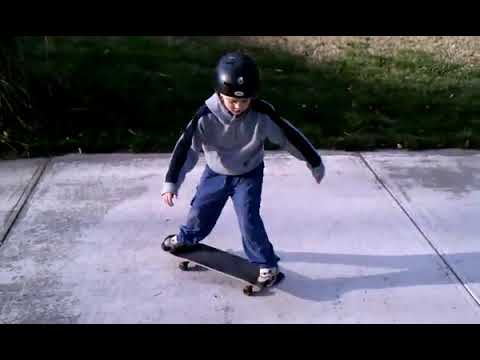The image depicts a small boy, likely around four or five years old, standing on a skateboard positioned on a gray cement sidewalk. The sidewalk has visible lines splitting it into squares. The background features shadows and patches of grass, with the scene somewhat obscured in darkness. At the top and bottom of the image, there is a black border framing the photograph. The boy is wearing blue jeans, white sneakers, and a long-sleeved gray sweatshirt that might be a hoodie. He dons a black helmet with a logo on it, and his arms are extended to each side as he looks down at the skateboard.